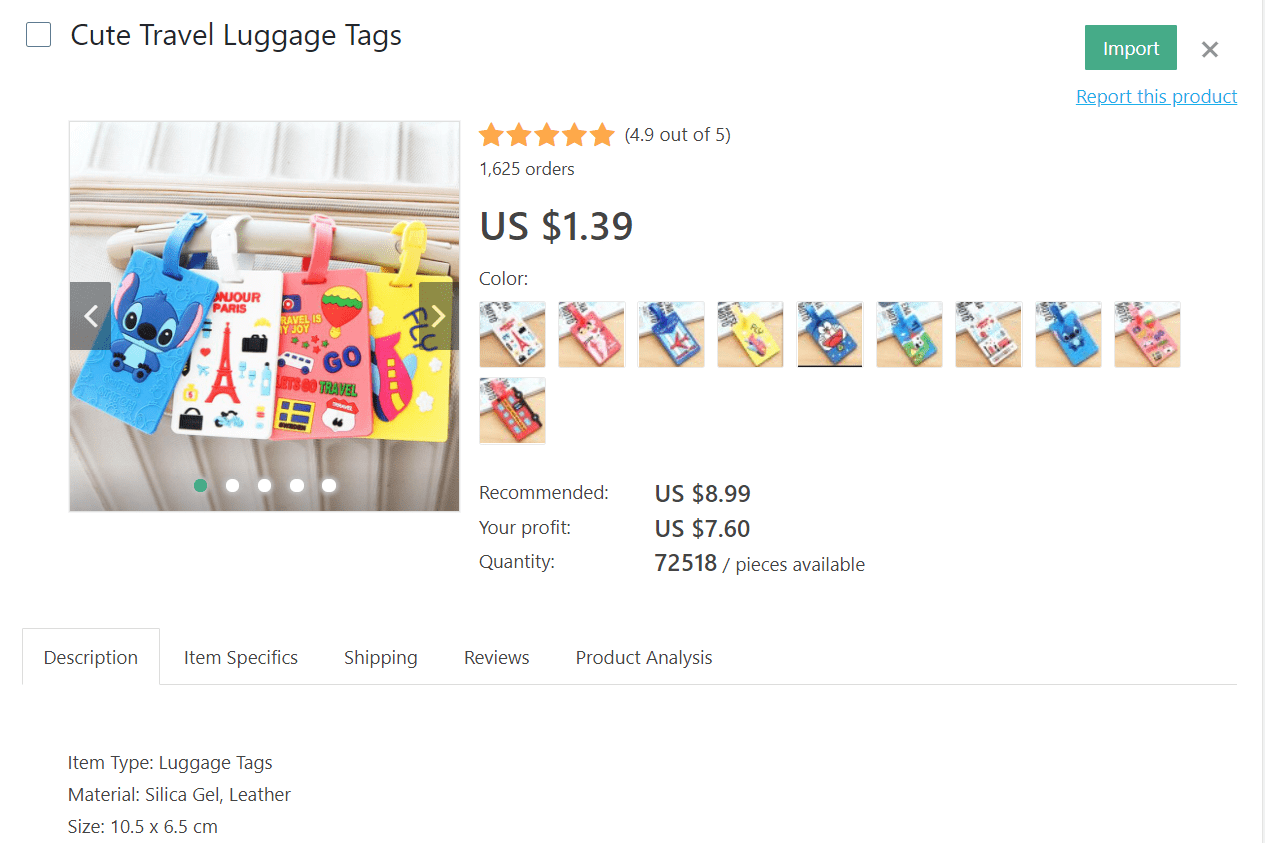Caption: 

This image appears to be a listing for cute travel luggage tags on eBay. Starting at the top left, there's a checkbox labeled "Cute Travel Luggage Tags," which is currently unchecked. Below this, a photograph showcases the tags attached to a piece of luggage. The tags are themed, featuring designs such as Lilo and Stitch, Paris, "Let's Go Travel," and an airplane with the word "Fly."

To the right of the image, the item is rated 4.9 out of 5 stars, and all five stars are highlighted in gold. The listing shows that 1,625 orders have been placed. These tags are priced at $1.39 each. In the top right corner, there is an option to report the item, and a button for importing it from another country. The recommended retail price is listed as $8.99, with a stated profit of $7.60 per tag, and there are 72,518 pieces available in quantity.

Below this section, there are tabs for more details, including "Description," "Item Specifics," "Shipping," "Reviews," and "Product Analysis."